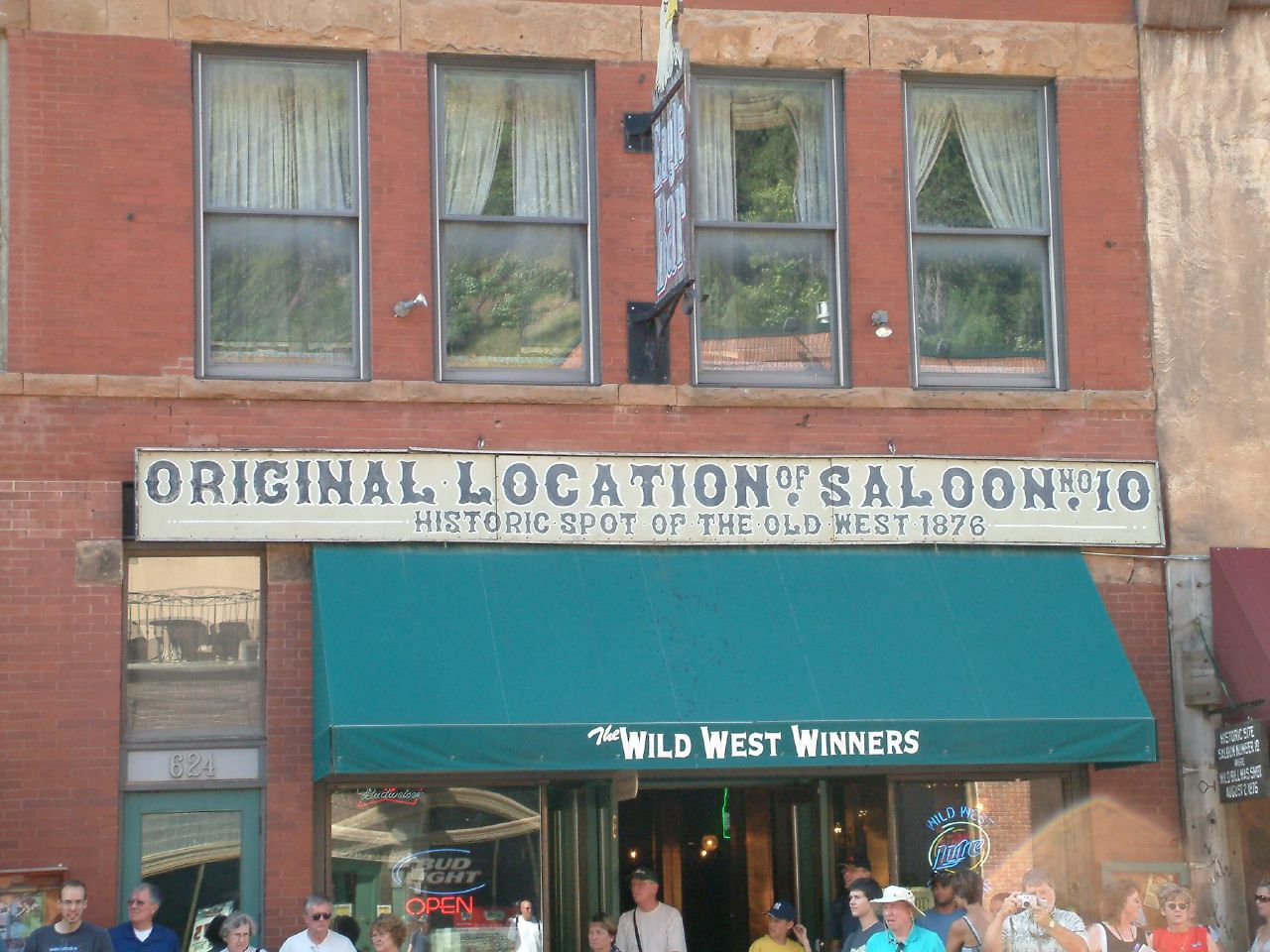The image depicts an outdoor daytime scene in front of a historic bar-type restaurant named "The Wild West Winners," located in a two-story red brick building. The building features a green awning with the establishment's name prominently displayed. Above the awning, an old, tan-colored sign with faded blue letters reads, “Original location of Saloon Number 10. Historic spot of the Old West 1876.” The upper floor of the building has four large rectangular windows adorned with curtains at the top. 

At street level, under the awning, several glass windows are visible, one of which displays a Bud Light neon sign indicating that the bar is open. There is another neon sign on the opposite side of the entrance. The front door of the establishment appears to be open. In front of the building, a crowd of people, including tourists and a few children, are standing. Many of them are wearing t-shirts and hats, suggesting warm weather. One man in the group is seen holding a camera, capturing a photograph. The people seem to be casually gathered, possibly waiting for an event or simply enjoying the historic ambiance of the location.